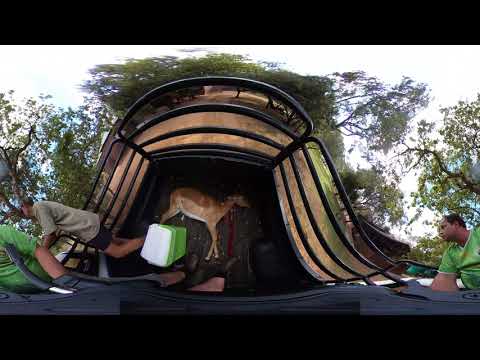This horizontally aligned, rectangular image with thick black borders on the top and bottom captures an outdoor scene during the daytime. The upper portion of the image showcases a sky filled with white clouds, with a tiny bit of blue visible on the upper left side, partially framed by some trees. We're looking down into the bed of a black pickup truck, which has metal railings made of four horizontal pipes on its sides.

In the center of the truck bed lies a dead doe with a stream of blood visible from its neck. Adjacent to the deer, toward the left side, there is a green and white cooler. Positioned around the truck bed are three individuals. On the far left, we see part of a person’s arm and sleeve, clad in a short-sleeved green shirt. Next to them stands another male, wearing a short-sleeved brown shirt and black shorts, with short brown hair. On the right side of the image, there is a man in a green v-neck t-shirt, with short brown hair, looking towards the left.

Surrounding the pickup truck, the ground is brown dirt, and beyond that, there are densely packed trees with a gray sky above them. This image seems to depict a moment after a hunting trip, with the individuals organizing the truck bed.